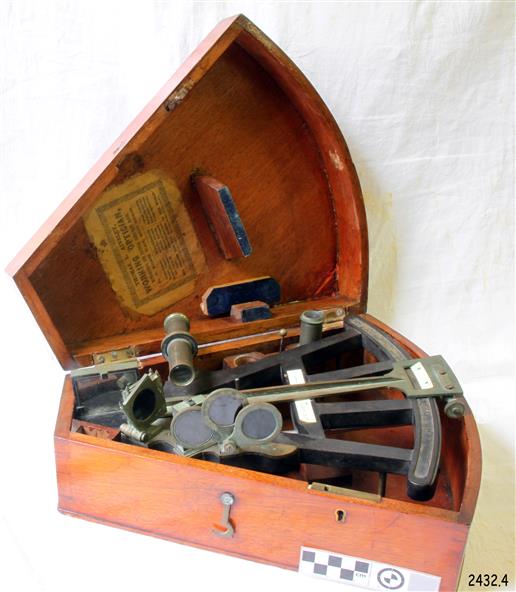The photograph depicts an old wooden case made of walnut-like wood, with visible cracks and scuff marks, indicating its age. The shape of the case is peculiar, vaguely fan-shaped, featuring a tapered triangular base that widens and rounds outward. The case is open, revealing two gold or copper-colored hinges at the back and a keyhole with a latch for securing it. Inside the case, there is a complex metal instrument, which appears to be a sextant, although it has additional lenses and features that might suggest otherwise, including a slider and telescope-like components. The instrument is primarily black with some parts showing an oxidized greenish bronze hue. The inside of the lid has an old, rectangular yellowish-brown label that reads "Working Optician." Positioned directly beneath the box, resting on a white fabric sheet that serves as both the background and bottom, is a paper tag in the lower right-hand corner with the black print "2432.4."